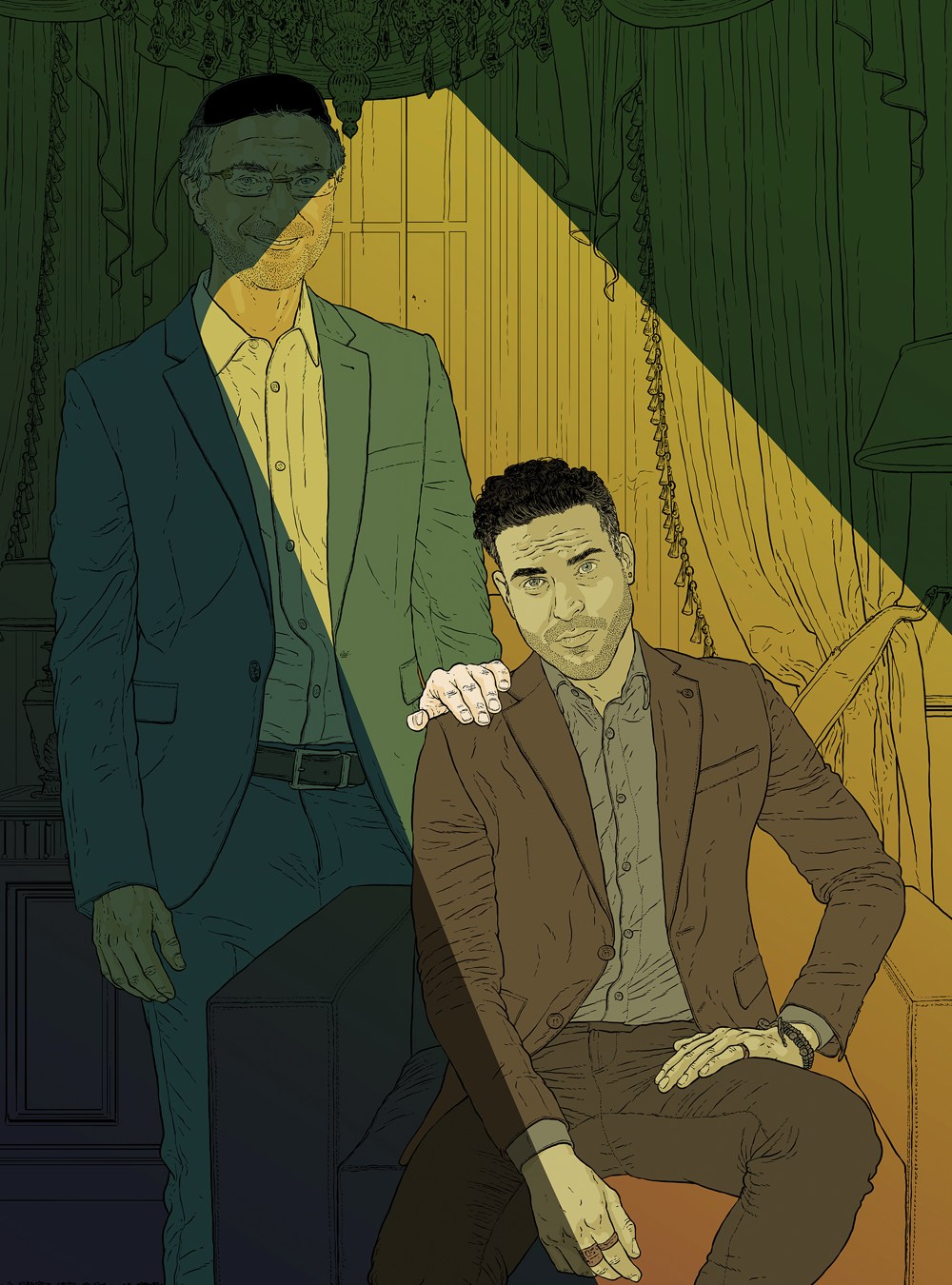The image is a hand-drawn, cartoonish depiction of two men in a dimly lit room with a distinct yellow background. The scene shows a man sitting down, wearing a brown suit with a gray buttoned-up shirt underneath, brown pants, and rings on his right hand. He has black hair and a stubble beard, and his left wrist bears a brown bracelet. His pose is relaxed, with one hand on his hip and the other resting between his legs, and he gazes directly at the viewer.

Standing behind him, a slightly older man with glasses rests his left hand on the seated man's shoulder. This older man, who has black hair speckled with gray, is dressed in a bluish-green suit with a white button-up shirt. The background features ornate details like curtains and lamps, with shadows indicating a darker ambiance, except for a beam of light streaming into the scene, casting an illuminating glow on the seated man and partially on the standing man. The room is detailed with thin black lines, enhancing the cartoonish yet intricate style of the drawing.